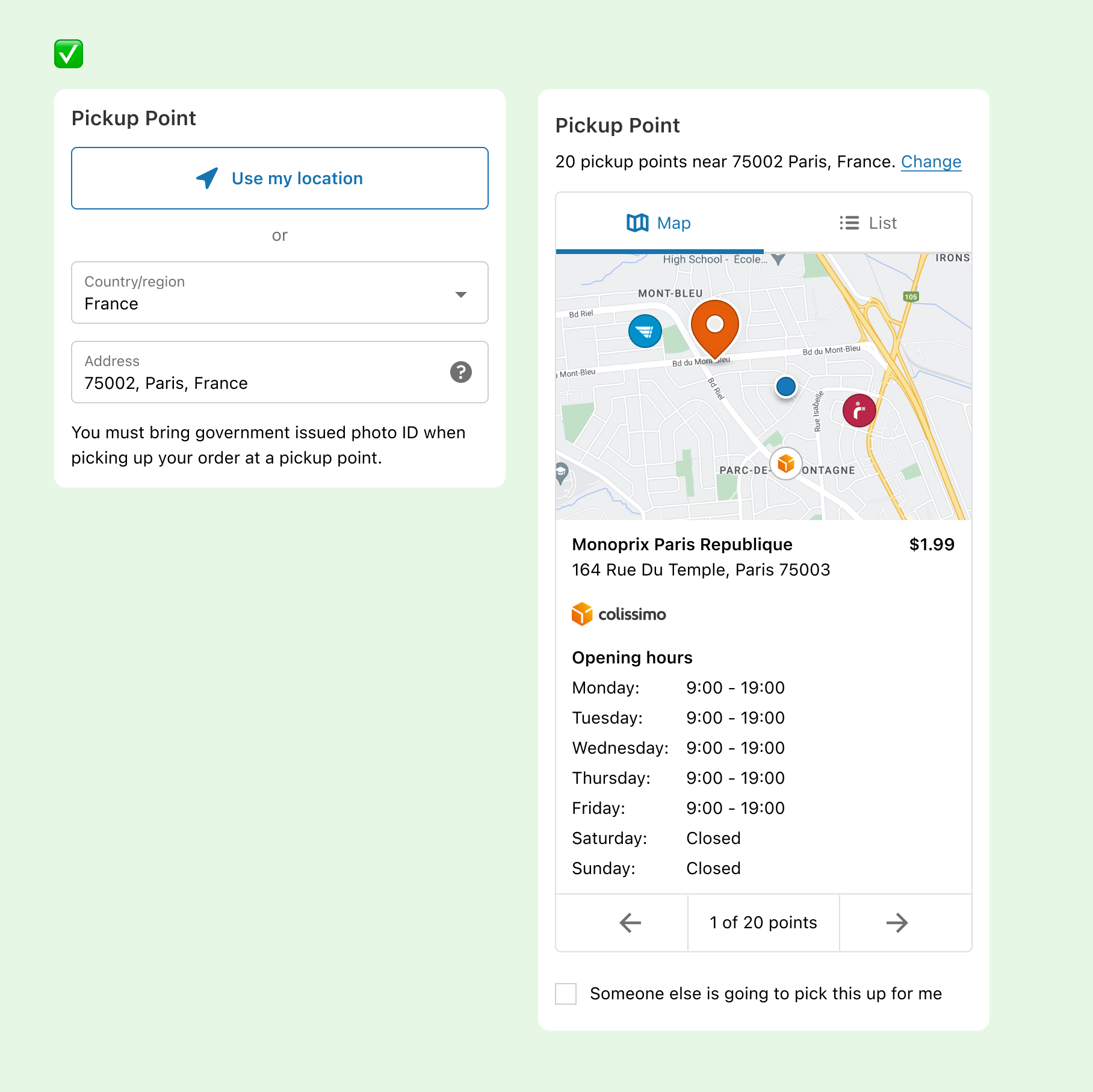The image features a user interface with a primarily black and light blue background. In the top-left corner, there is a small green square adorned with a white checkmark. Below this, a white square, measuring approximately three inches by three inches, displays the text "Pick Up Point" in black in its top-left corner. The square is bordered on its top by a thin blue line and contains a white tab that reads "Use My Location," accompanied by an arrow pointing up to the right. Beneath this tab, the word "or" appears in small black letters.

Further down, another tab labeled "Country/Region" is present, specifying "France." Below that, there is a section for entering an address, followed by a notice in smaller fonts advising, "You must bring government-issued photo ID when picking up your order at a pick-up point."

Adjacent to this, on the right, there is a taller but equally wide white background feature with "Pick Up Point" written at the top. Underneath, it states, "20 pick up points near the address you choose." This section includes a blue tab with a map icon labeled "Map," and a black tab with a list icon labeled "List."

Below this, there is a visual representation of a map. The map has a blue background, with white denoting regular streets and yellow representing interstates. A prominent orange location marker with a white center is displayed, along with icons for various amenities like restaurants. At the bottom of the map, there are details in black text regarding specific places, their prices, and opening hours, specifying the days they operate and their exact opening and closing times.